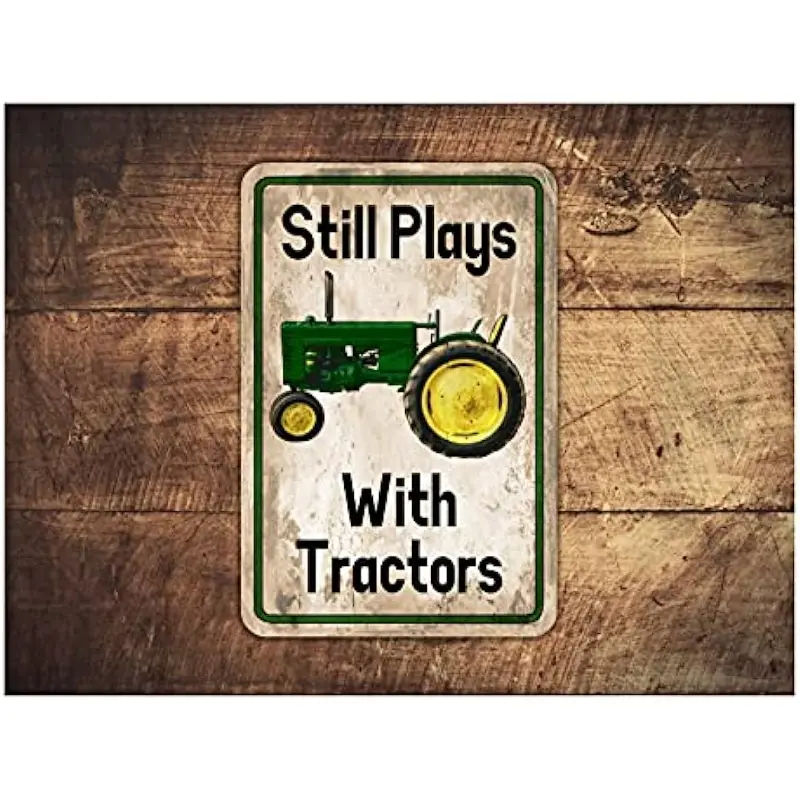The image showcases a detailed photo of a sign affixed to a distressed, dark brown wooden wall composed of horizontally aligned slats, complete with visible etches and knots. The sign, similar in material to a metal street sign, has a white background framed by a distinct green border. Positioned centrally on the sign is a profile of a green tractor with one large yellow-rimmed back wheel on the right and a smaller yellow-rimmed front wheel on the left, all set against the backdrop of the wooden slats. Above the tractor, in bold black block letters, the sign reads "Still Plays," and below it, "With Tractors," emphasizing the playful nature of its message. The sign's overall appearance hints at a weathered, rustic aesthetic, reminiscent of a whimsical gift shop plaque meant for someone with a fondness for farm life or quirky humor.